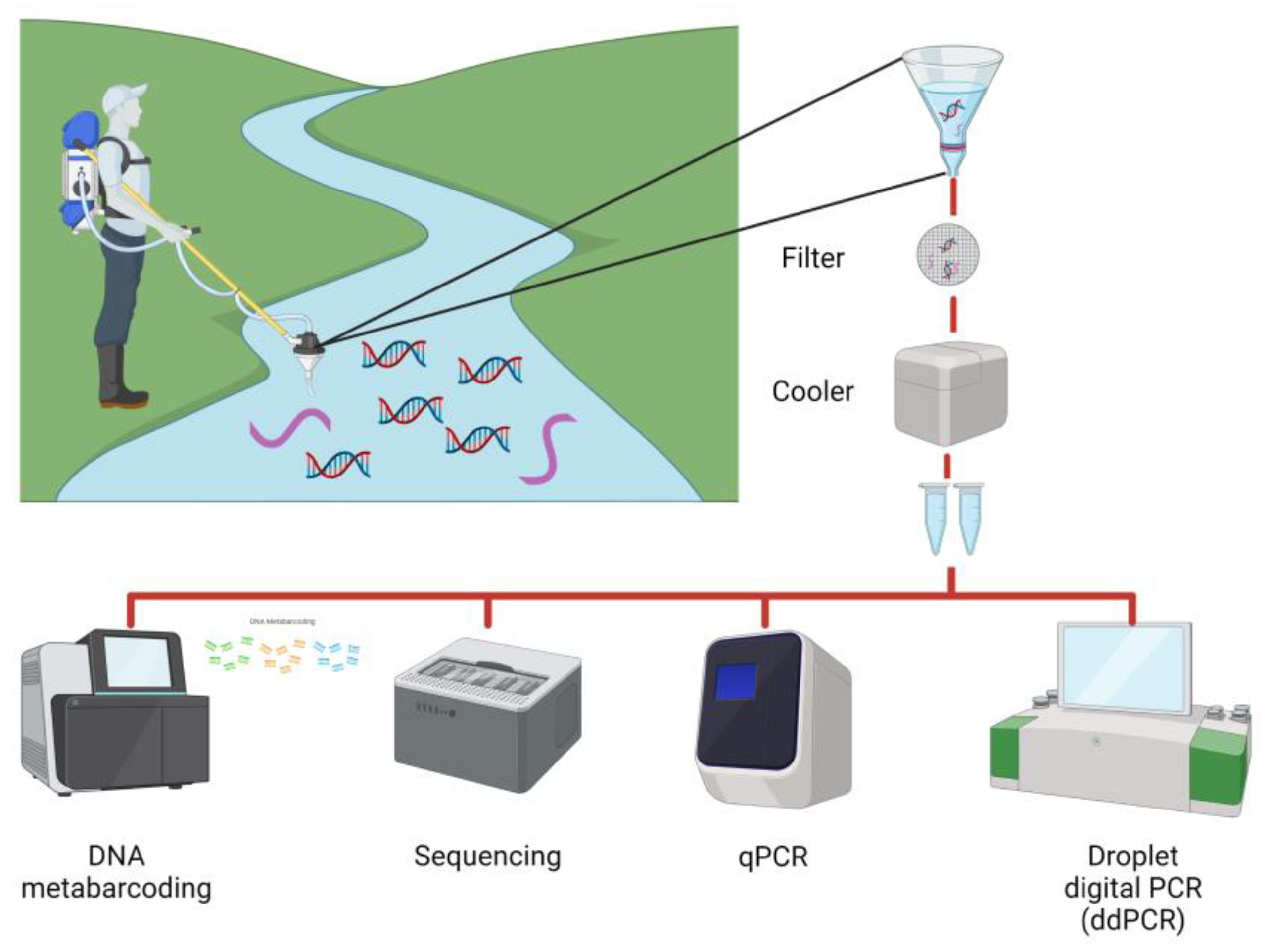The image is an intricate animated diagram set against a solid white background. At the top left, a large rectangular illustration depicts a hilly green field bisected by a stream or waterway. A man stands on the left bank, dressed in a white cap and shirt, with blue pants and black boots. He has a backpack-style apparatus, holding a yellow hose dipped into the water. The apparatus is white with blue accents, suggesting it's designed for ecological sampling.

To the right of this scene, a series of labeled components are connected by lines to the apparatus. These include a cone-shaped filter, a square cooler, and vials presumably containing water samples. Below this, a horizontal red line runs across the image, with vertical lines pointing down to various laboratory machines. These machines, detailed with labels, are arranged from left to right: "DNA meta barcoding" attached to an object resembling a printer, "sequencing" on a square-shaped device, "qPCR" on a computer-like screen, and "droplet digital PCR (ddPCR)" on a monitoring device.

The image utilizes a color palette primarily of green, blue, black, purple, red, and shades of white, emphasizing both the natural environment and the scientific equipment. Overall, the diagram appears to depict a field-based ecological sampling process followed by laboratory analysis.